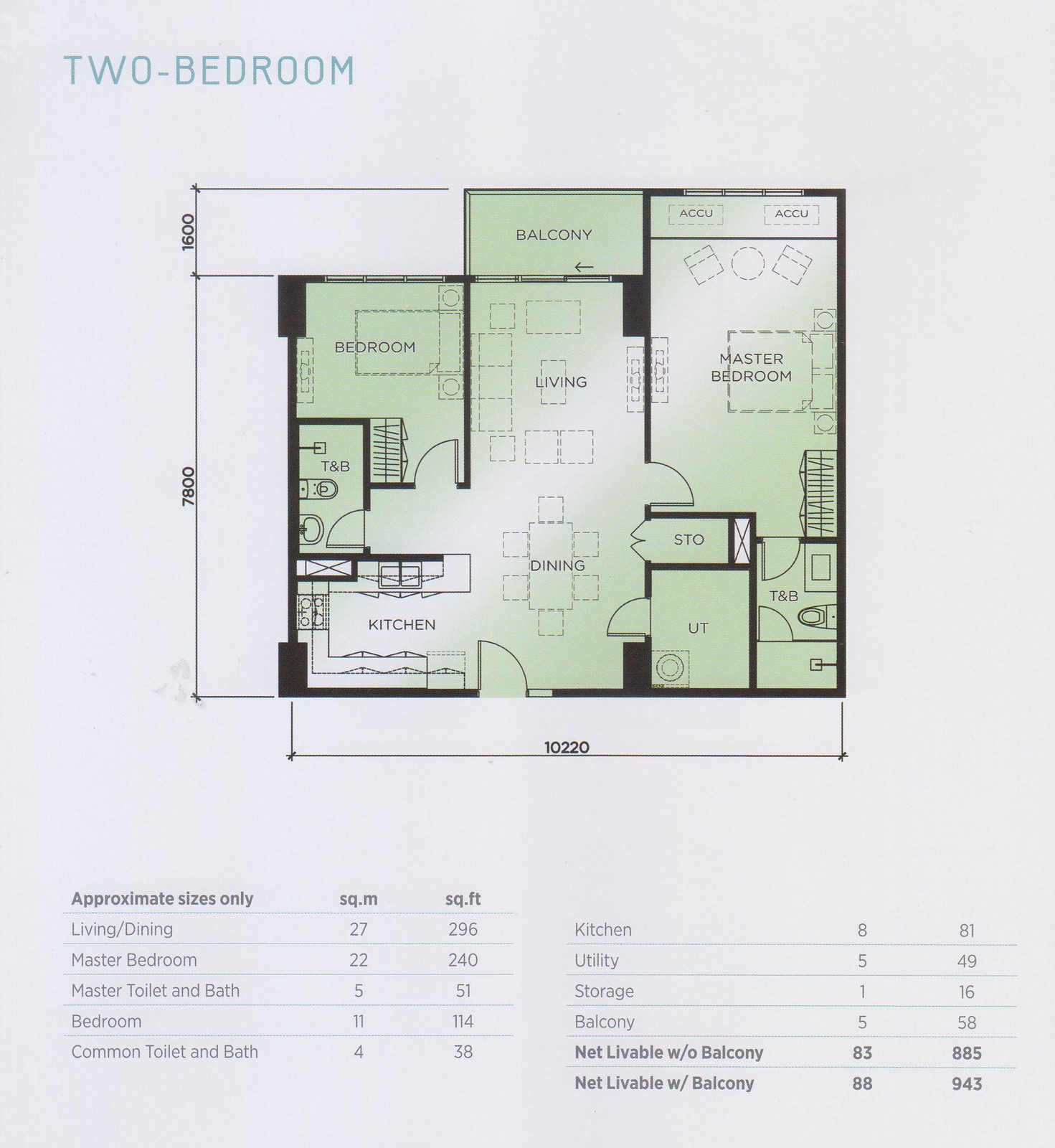Detailed Floor Plan of a Two-Bedroom Apartment

The image features a detailed floor plan of a two-bedroom apartment, prominently titled "TWO BEDROOM" in capital letters in the top left-hand corner. The diagram, rendered in a light green color, clearly delineates walls with thick black lines and includes various markings indicating the dimensions and layout of the space. Each room is labeled, and the layout includes dashed lines suggesting potential furniture placements.

Upon entering the apartment through the door situated in the center of the front wall, one immediately encounters the U-shaped kitchen to the left. Directly ahead is the dining area, which transitions seamlessly into the living area located behind it. To the left of this transition zone lies a corridor leading to the common bathroom. Adjacent to the living room, on its right-hand side, is the first bedroom, sharing a wall with the living room. Further right, the master bedroom is positioned, also adjoining the living space, and it includes a private bathroom at its front.

Additionally, the floor plan provides detailed measurements of each area in both square meters and square feet as follows:
- Living/Dining Area: 27 square meters (296 square feet)
- Master Bedroom: 22 square meters (240 square feet)
- Master Bathroom: 5 square meters (51 square feet)
- Second Bedroom: 11 square meters (114 square feet)
- Common Bathroom: 4 square meters (38 square feet)
- Kitchen: 8 square meters (81 square feet)
- Utility Area: 5 square meters (49 square feet)
- Storage: 1 square meter (16 square feet)
- Balcony: 5 square meters (58 square feet)

The bottom section of the floor plan features additional information, noting the net livable area as 83 square meters (885 square feet) without the balcony, and 88 square meters (943 square feet) including the balcony.